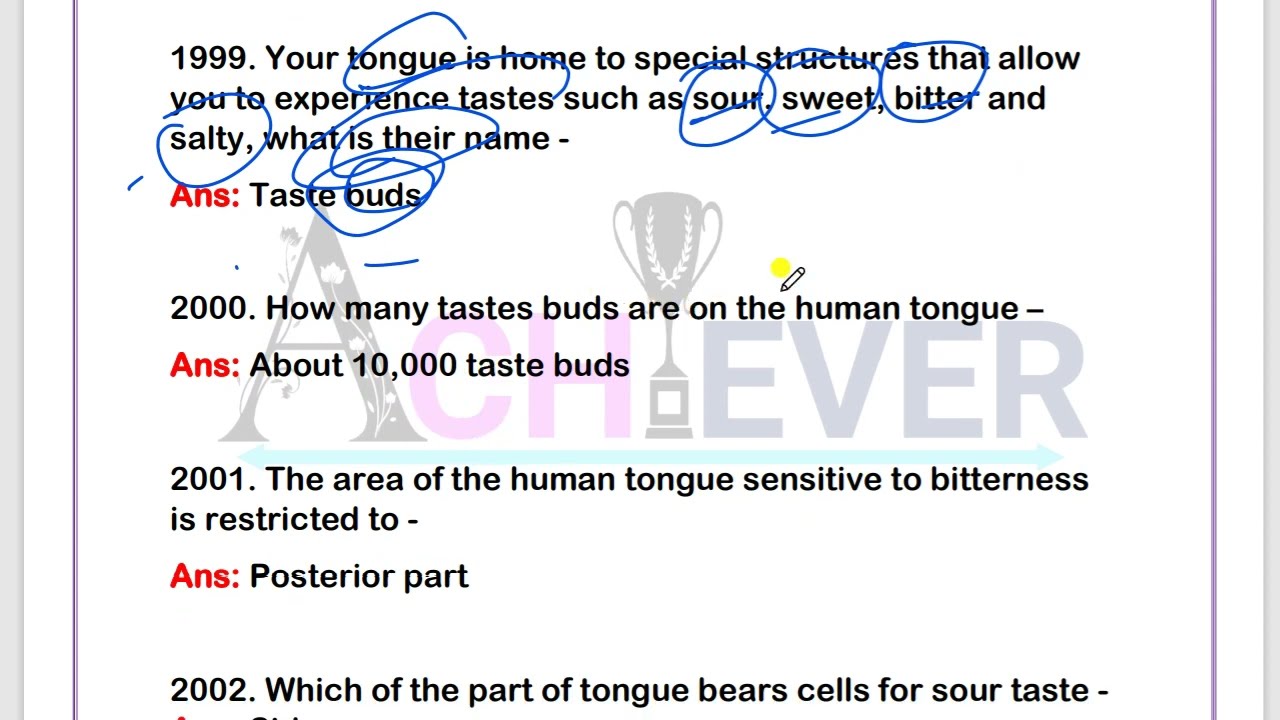The image features a white background with the word "Achiever" in ornate lettering, where the 'A' is notably larger and the 'i' is represented by a trophy icon. This suggests it might be styled for an educational or motivational presentation, possibly a graphic for a PowerPoint slide or a section of a study guide. The content appears to be formatted in a question-and-answer style, with questions and answers listed chronologically from 1999 to 2001. Each question is printed in black text, with the answer, prefixed by "ANS:" in bold red lettering.

Additionally, hand-drawn blue circles and scribbles indicate digital notation, possibly for annotation or correction. The repeated questions relate to the human tongue’s functionality and structure, mentioning specific details like taste buds and their quantities, and the regions of the tongue sensitive to different tastes. Keywords such as "tongue," "structures," "bitter," "sweet," "sour," "salty," and "buds" are circled, emphasizing important concepts, hinting at this being a detailed study guide or medical journal extract, providing both educational and detailed scientific information.